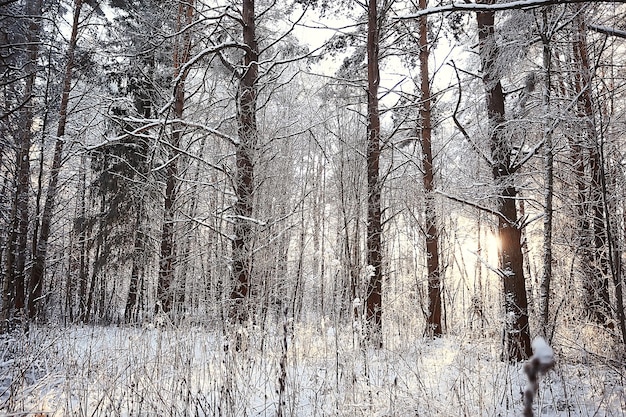This professional color photograph captures a stunning winter scene in a dense forest. The image, taken in a landscape orientation, showcases tall, mature trees, some of which are likely pine or cypress, and others are deciduous trees stripped of their leaves. Their heights reach an impressive 50 to 60 feet. The ground is blanketed in a thick layer of snow, though it appears walkable, and the underbrush is sparse, consisting mainly of bare branches, dead grass, and thin, twiggish plants. The scene is permeated with a quiet, serene atmosphere. The sun is seen peeking through the lower right side of the image, either just rising or setting, casting a soft light that gently illuminates the snow-covered landscape. The sky is overcast with white clouds, adding to the stark, cold beauty of the winter forest. There are no signs of human presence, structures, or animals in the scene, allowing the viewer to fully immerse in the undisturbed, natural beauty of this wintry forest landscape.